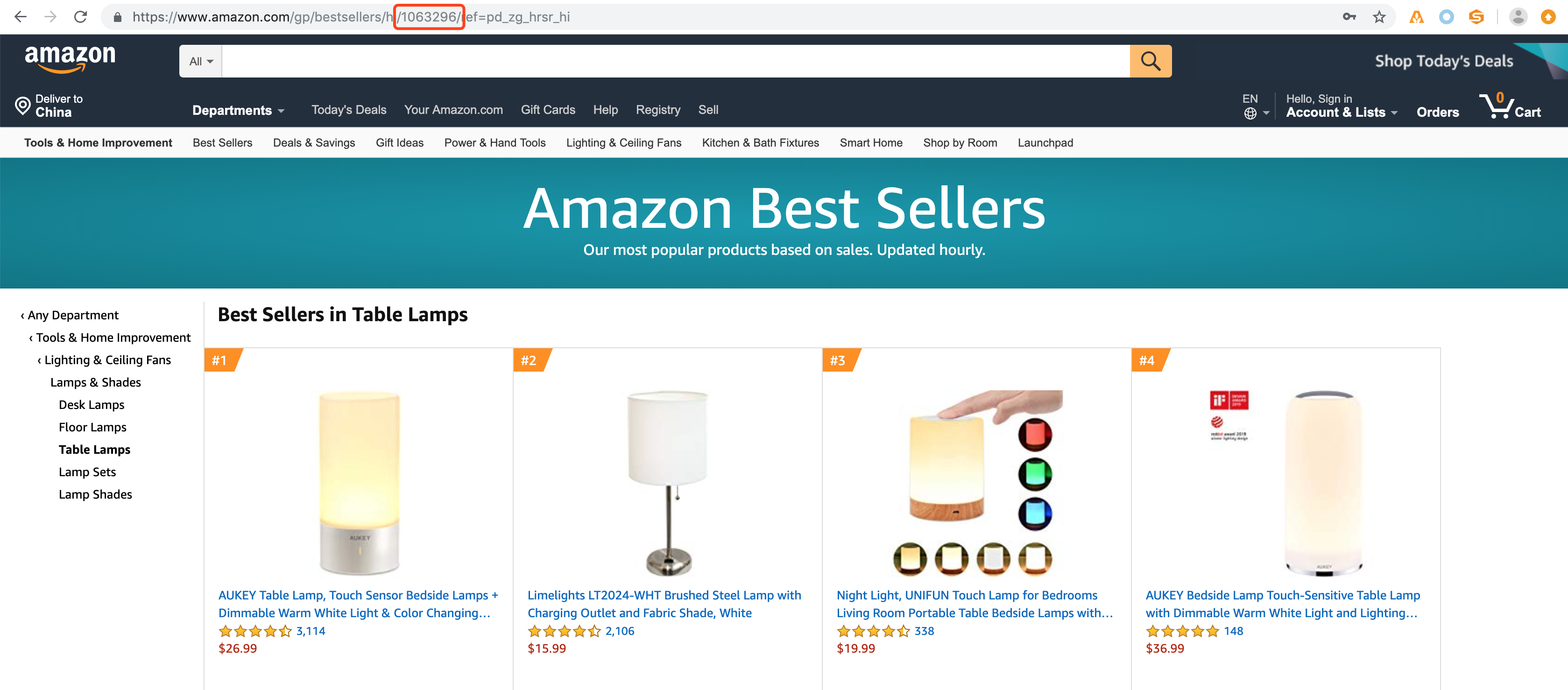The image is a screen capture of the Amazon.com shopping website, displaying a section for bestselling items. The webpage has a white background with key horizontal sections highlighted in black and green. At the top, the black bar features the Amazon logo in white with an orange arrow, positioned in the upper-left corner. Adjacent to the logo is a white search bar with an orange search button on its right side.

Below the black bar, a prominent green rectangular banner spans horizontally, displaying the text "Amazon Bestsellers" in large white font. Underneath this green banner, the page continues with a white background showcasing four images of various table lamp designs. Above these images, aligned to the left above the first lamp, is the heading "Bestsellers in Table Lamps" indicating that the featured items are popular choices in this category.